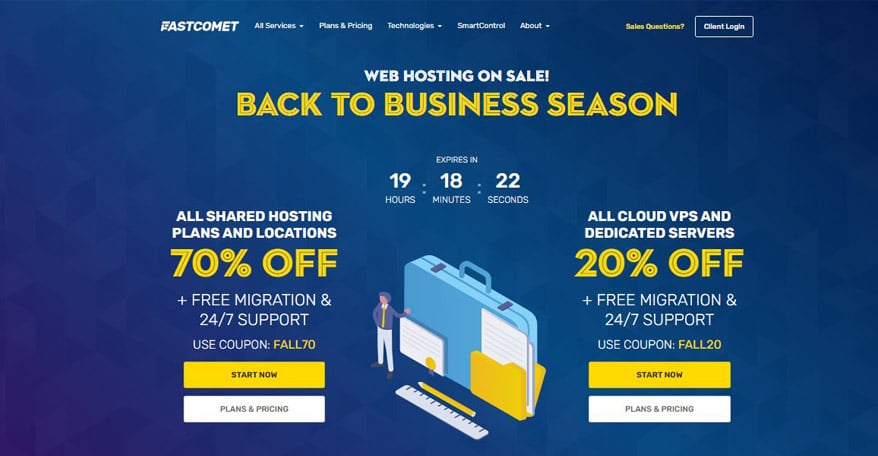This screencap depicts the homepage of the website "Fast Comet," which specializes in web hosting, servers, and cloud VPS services. At the top, a centrally positioned navigation bar displays options such as "Services," "Plans & Pricing," "Technologies," "Smart Control," and "About." Additional features on the navigation bar include a "Sales Questions" option and a "Client Login" button.

Directly below the navigation bar, a bold header announces a "Web Hosting on Sale" event with the tagline "Back to Business Season." A countdown timer prominently displays the remaining time until the sale expires, currently showing 19 hours, 18 minutes, and 22 seconds.

The focal graphic beneath the header features a clipart image of a briefcase accompanied by a small figure and various scattered papers. This graphic is flanked by text and buttons providing details on the discount percentages, available coupon codes, and actionable buttons labeled "Start Now" and "Plans & Pricing," encouraging immediate engagement with the available offers.